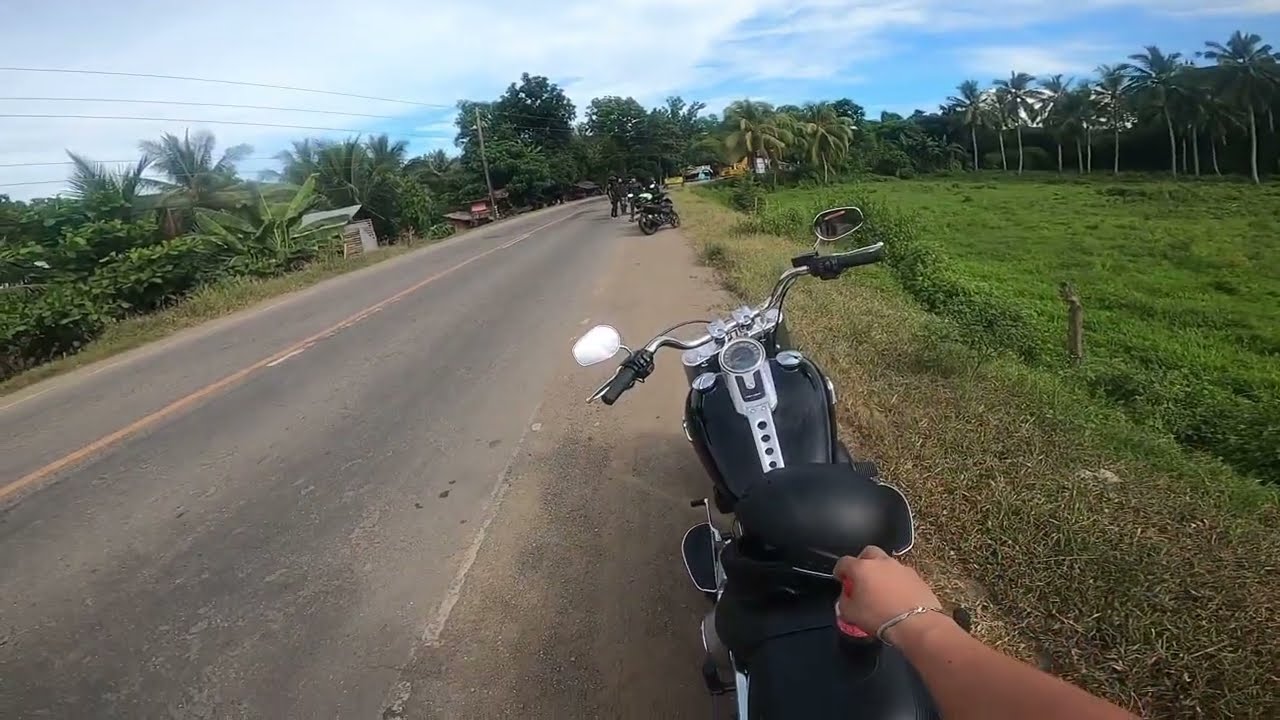The image captures a daytime scene with partially cloudy skies. The main focus is a black motorcycle with silver trim positioned on the right side of the road, which runs diagonally from the bottom left toward the top center of the frame. A person, likely a woman wearing a bracelet, has her arm extended toward the motorcycle, holding a pink object. The road is flanked by lush vegetation, with tropical trees and palm trees visible both to the left and right, and a grassy area leading into a ditch on the right. In the background, approximately 30 to 50 yards away, there are more motorcycles and people dressed in black, standing by the road's shoulder, though they appear blurry due to the distance. The left side of the road also features palm branches, other trees, some shacks, and telephone wires. The scene suggests a Southern or tropical locale, enriched with vibrant greenery and a laid-back atmosphere.